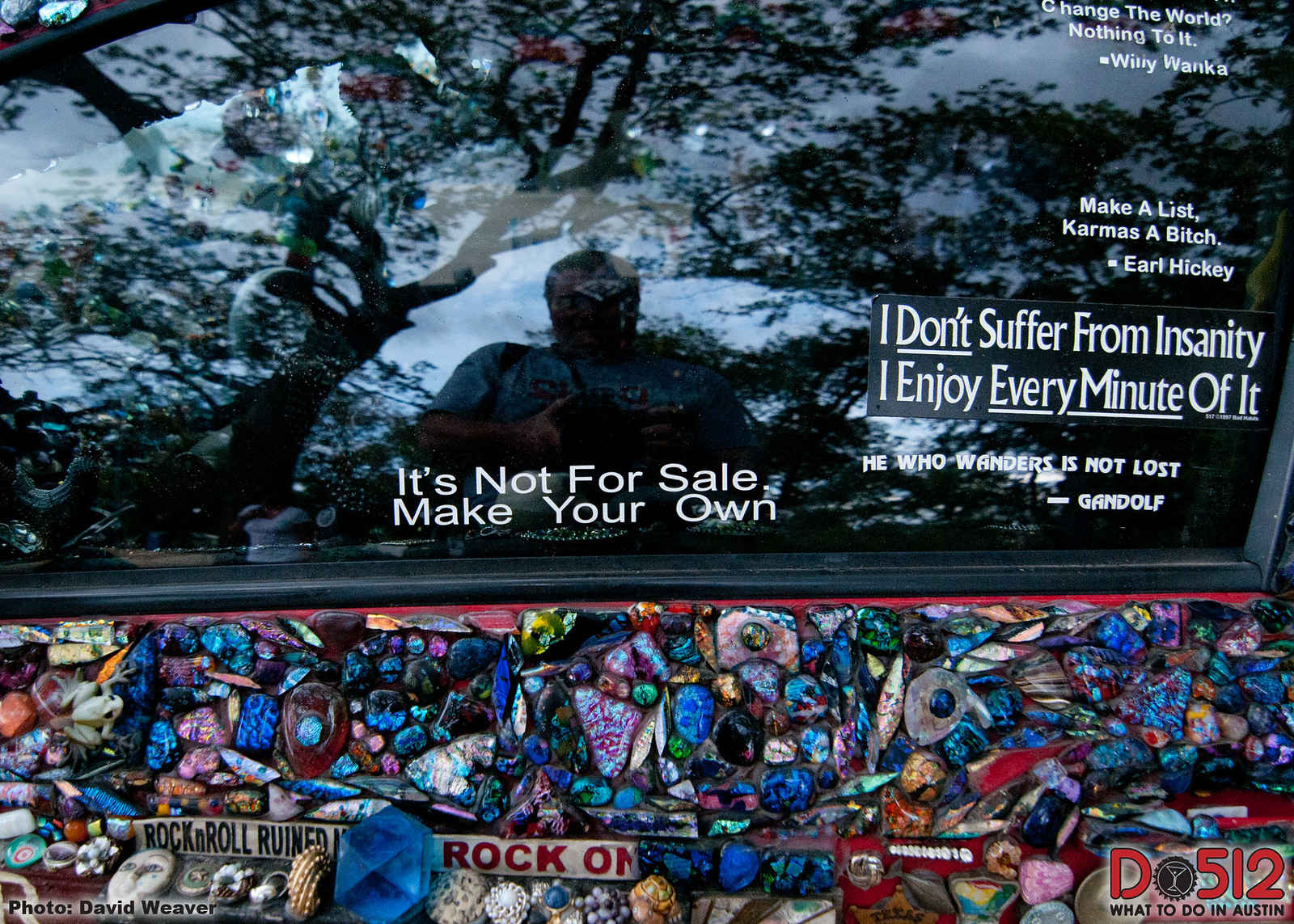This image captures the back of a uniquely decorated vehicle, focusing on the rear windshield and the area immediately below it. The bottom portion of the car is intricately adorned with a multitude of colorful stones, possibly including some jewels and shells, forming a detailed and elaborate arrangement. Among these decorative stones are red text labels stating "Rock and Roll Ruined" and "Rock On." In the bottom left corner, the image credits "Photo by David Weaver," while the bottom right corner features a logo saying "D512 What to Do in Austin."

The rear windshield of the vehicle is loaded with various bumper stickers with white text on black backing, making them stand out vividly. The stickers convey a mix of whimsical and motivational messages such as "It's not for sale, make your own," "Change the world, nothing to it" attributed to Willy Wonka, "Make a list, karma's a bitch" credited to Earl Hickey, "I don't suffer from insanity, I enjoy every minute of it," and "He who wanders is not lost" attributed to Gandalf. The reflection of the person taking the picture is faintly visible in the window, adding a human element to this eclectic and vibrant visual display.